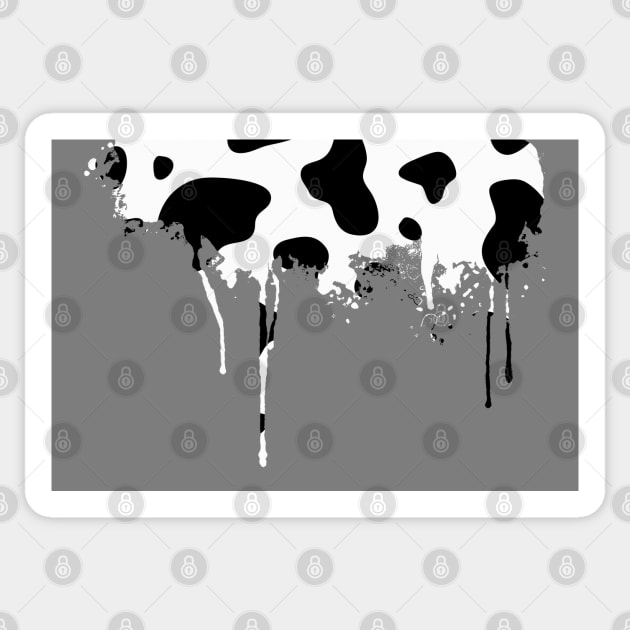This image features a rectangular frame with rounded corners, predominantly filled with a dark gray background. At the top of the frame, a striking cow print—characterized by black patches on white—drips downwards, creating a splatter effect that extends toward the bottom of the image. Encasing the frame is a white bevel, distinguishing it from the rest of the background. Overlaying the entire image, including the cow print and the gray background, is a semi-transparent watermark comprised of padlocks arranged in a diagonal grid pattern, reminiscent of combination locks used in school lockers. This watermark adds an additional layer of texture across the image, providing a sense of depth and complexity.